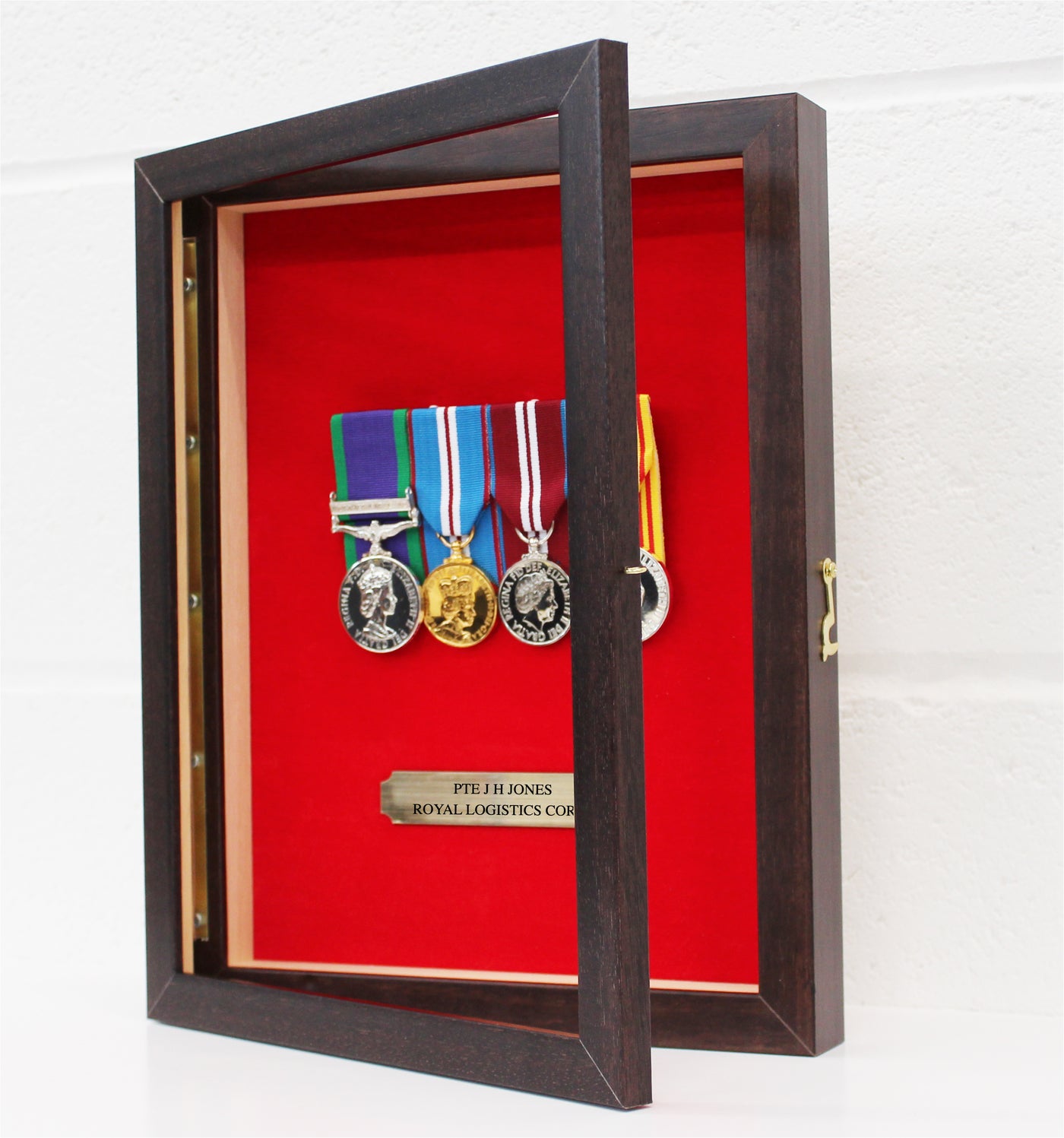The image portrays a wall-mounted, glass-fronted display case made of brown wood with gold metal hinges and a lock. The case has a red felt background and contains four military medals, each suspended by their respective ribbons. The medals are arranged in a row from left to right. The first medal, silver with an embossed face, hangs from a dark blue ribbon with green edges. The second medal, gold in color, is attached to a blue ribbon with a white and red stripe. The third medal is silver, accompanied by a red ribbon with white lines. The fourth medal has a yellow and red ribbon, though only partially visible. Below the medals, a gold plaque reads: "PTE JH Jones Royal Logistics Corp." The case is mounted on a white wall, further emphasizing the distinguished display.